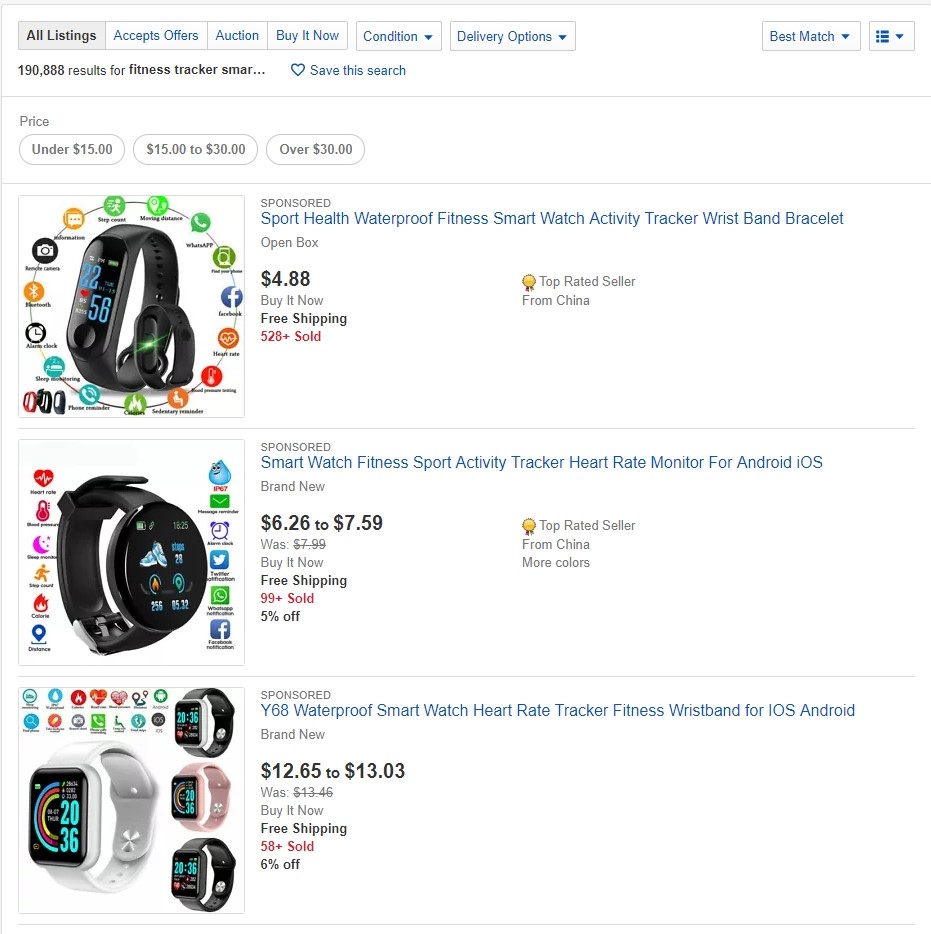Search results displaying a variety of smart watches and fitness trackers are presented, possibly from eBay based on the layout and search options available at the top: "All Listings," "Accepts Offers," "Auction," "Buy It Now," "Condition," "Delivery Option," and "Best Match." A total of 190,888 results for "fitness tracker smart watch" are shown, with price filter buttons available for under $15, $15 to $30, and over $30.

1. **Sport Health Waterproof Fitness Smart Watch Activity Tracker Wrist Band Bracelet**:
   - **Price**: $4.88
   - **Shipping**: Free, from China
   - **Sales**: 528 sold
   - **Features**: Includes a photograph of two watches, highlighting the beam on the underside which likely indicates pulse-check functionality. Social media icons are arranged in a circle around the image.

2. **Smart Watch Fitness Sport Activity Tracker Heart Rate Monitor for Android, iOS**:
   - **Price**: $6.26 to $7.59
   - **Features**: The listing shows social media icons on both the right and left sides of the product image, along with regular activity icons. The watch is compatible with both Android and iOS.

3. **Y68 Smart Waterproof Smart Watch Heart Rate Tracker Fitness Wrist Band for iOS, Android**:
   - **Price**: $12.65 to $13.03
   - **Features**: The image displays several wristbands, including colors like white, black, and silver. The center features a prominent, larger-sized wrist band. The display seems cluttered with various icons.

Overall, users are shown a diverse selection of affordable fitness trackers and smart watches, highlighting features such as heart rate monitoring and waterproof functionality.